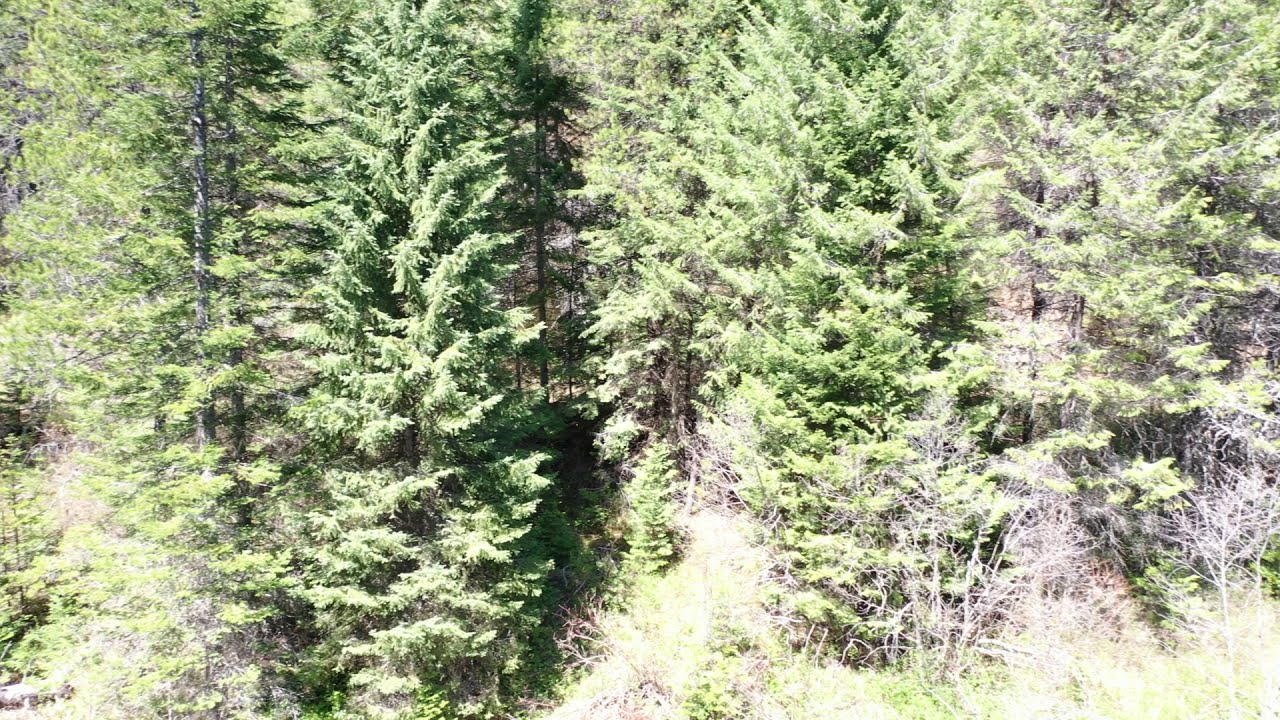The image depicts a sun-drenched, densely-packed forest captured from a top-down aerial view, likely taken by a drone or helicopter. The intense brightness from behind the camera results in a whitewashed effect, obscuring some finer details. Dominating the scene are very large trees, possibly fir or fern-like, resembling oversized Christmas trees standing approximately 60 feet tall. Among them are a few slender trees and some visible dead branches on the bottom right. The canopy is lush and green, with some patches of gray foliage, making it almost impossible to see through to the tree trunks, though a few are faintly visible at the center-bottom. The bright daylight accentuates the verdant leaves, giving them a vibrant, light green appearance, and saturates the entire scene with an abundant glow, emphasizing the thickness and beauty of this expansive, woodsy landscape.